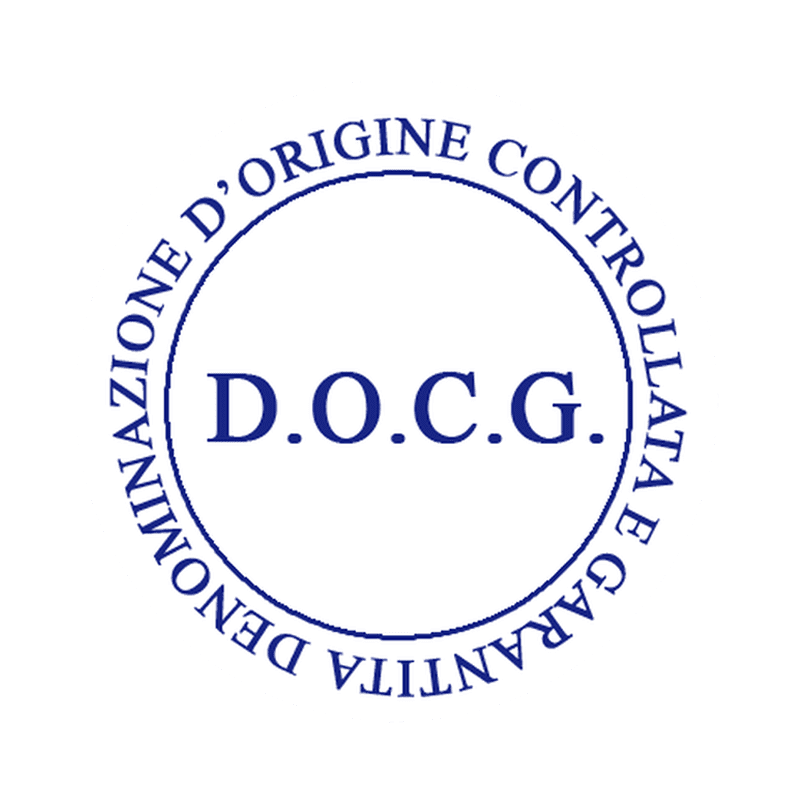The image depicts a simple yet elegantly structured circular logo, likely representing an organization or certification entity. The logo consists of a thin blue circular outline, within which the initials "D.O.C.G." are prominently displayed in a purplish-blue color, each letter separated by periods. Surrounding this inner circle, the phrase "Denominazione dell'origine controllata e garantita" is inscribed in the outer ring in a circular pattern. This phrase, Italian for "controlled and guaranteed designation of origin," indicates a certification standard, often associated with products of verified authenticity and quality, such as Italian wines. The design is clean, with all capitalized letters in both the central initials and the outer text, suggesting a formal and authoritative symbol, possibly computer-generated for precision.